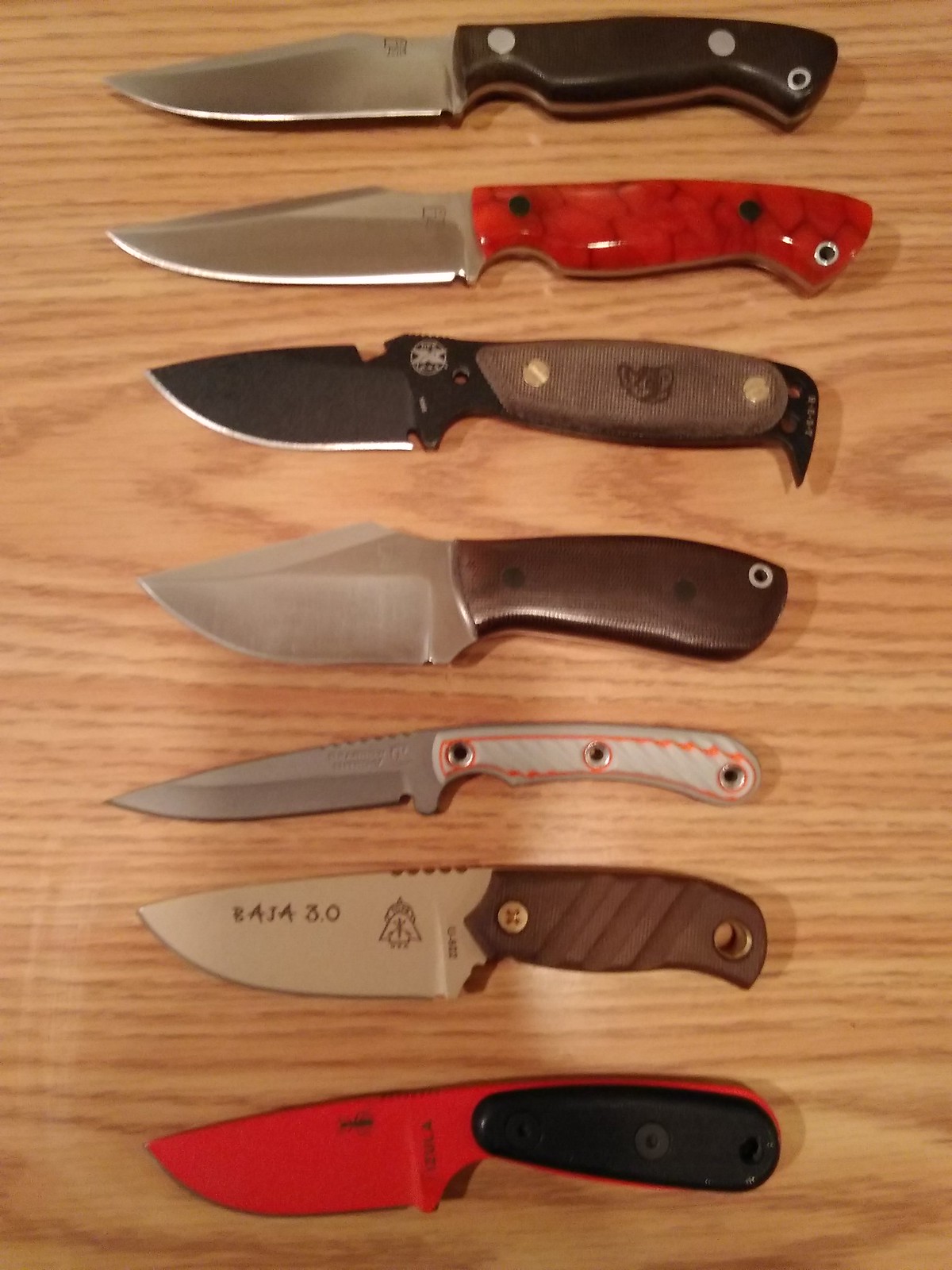This is a color photograph taken from a top-down perspective, showcasing seven diverse knives meticulously laid out on a wooden surface, likely a countertop. Each knife varies in both handle material and blade color. Starting from the bottom, the first knife features a striking red blade with a black handle. The next knife has a silver blade complemented by a brown handle marked with the text "Baja 3.0" and a large bronze screw, along with a small hole at the handle's base. Following is a smaller knife with a thin, silver blade and a white handle that has orange accents and three screw holes, perhaps indicating the handle was removed at some point. The fourth knife is handmade-like, featuring a short, stubbier design with a carved wooden handle and a plain metal blade. The fifth knife sports a symbol resembling an animal on its brown handle, with a distinctive black blade that has a silver or white edge. Next, an eye-catching knife has a red, marbled handle made from either acrylic or resin. The final knife in the lineup has a standard black kitchen knife handle secured with two metal studs, and a silver blade. The photograph, rich in detail and texture, seems to capture these knives possibly for display or sale, emphasizing their uniqueness and craftsmanship.